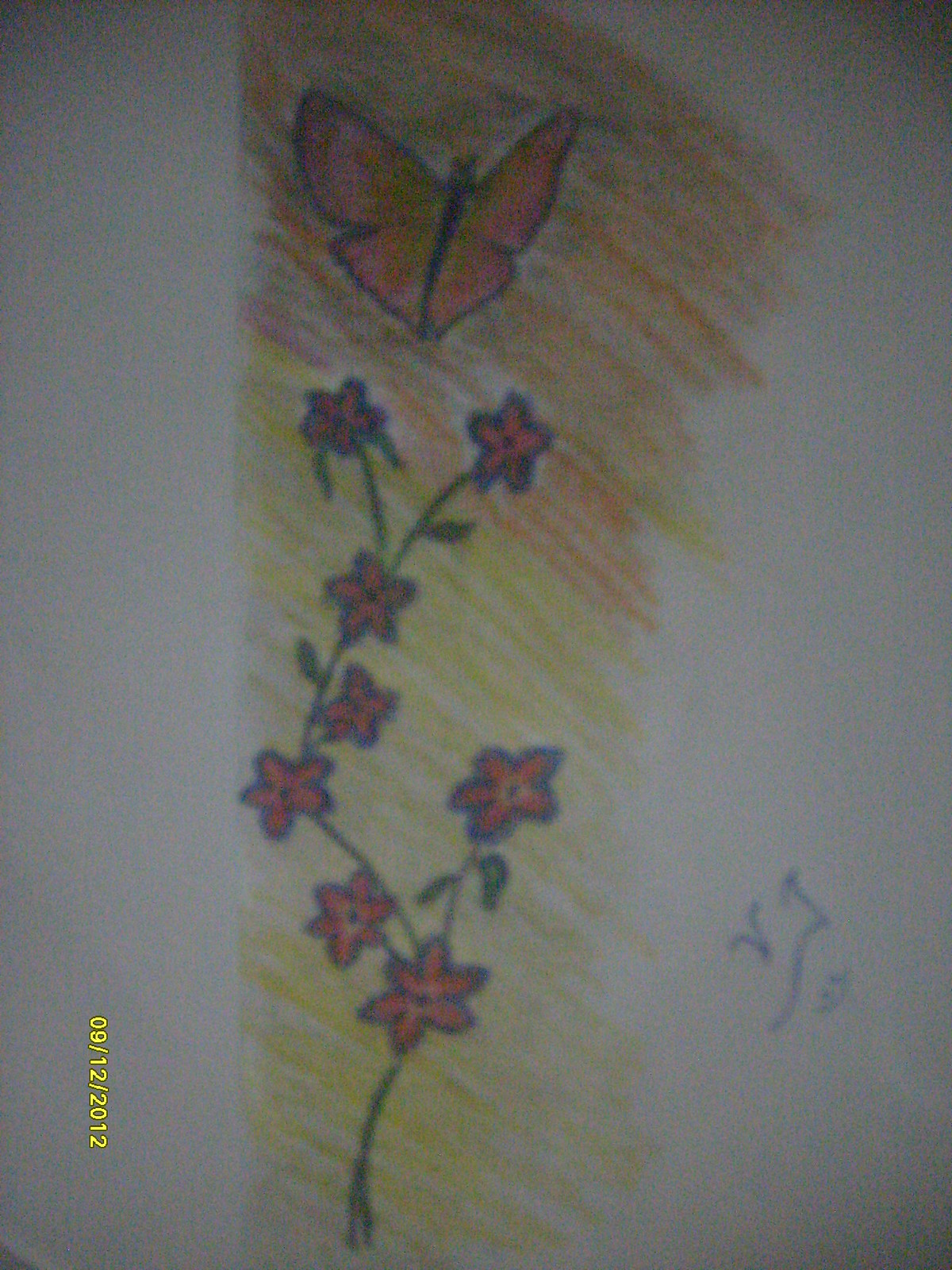The image is a crayon drawing on white paper of a vibrant scene featuring a butterfly and flowers. The background showcases a gradient that transitions from orange to yellow, creating a warm and inviting atmosphere. Centrally located and extending upwards, a long vine with green leaves is adorned with eight striking red and orange flowers. The red petals stand out prominently as they spiral up the vine. Hovering near the top right is a large butterfly with a black body and distinct red wings, which exhibit a yellow-to-red gradient. On the bottom left corner, there's yellow writing indicating the date 09-12-2012. Additionally, blue lines and the initials "VJ" are present in the lower right corner. The entire scene is both detailed and colorful, capturing the essence of a sunny day with its vivid use of colors and intricate design.